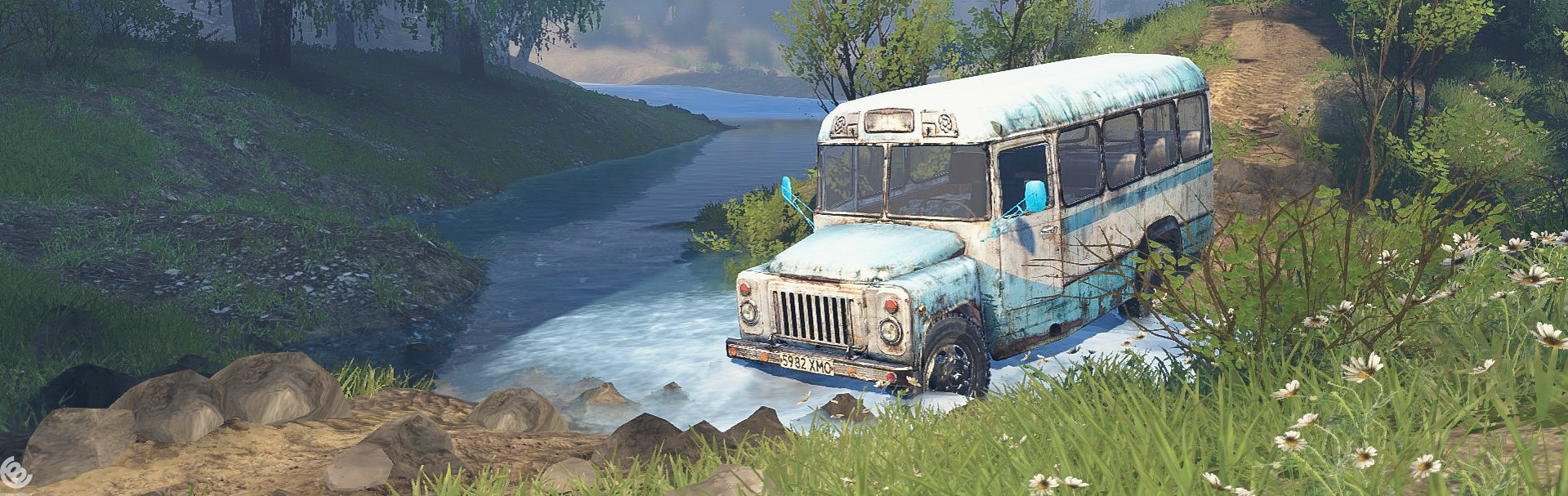This detailed computer-rendered image, reminiscent of a video game scene, depicts a serene outdoor setting featuring a u-shaped river with light blue and dark blue water, flanked by green grass-covered hills. A light brown dirt path in the foreground is lined with light gray boulders and rocks. Alongside this path, on the left side, tall green grass adorned with light white daisy flowers having brown centers contrasts against some emerging brown branches. A standout element in the image is a partially submerged, abandoned bus that straddles the bank and the water. The bus, predominantly white with blue stripes beneath its windows and along the front hood and lower margins, features four side windows, a windshield, side door windows, darker blue side mirrors, and large black tires. Positioned at an angle, the bus reveals a side profile view with its rear end resting on the grassy and dirt-covered ground. In the background, the river winds towards a lake, framed by distant mountains under a blue sky with clouds. The greenery includes weeds, shrubs, and several trees, completing this tranquil meadow-like scene.